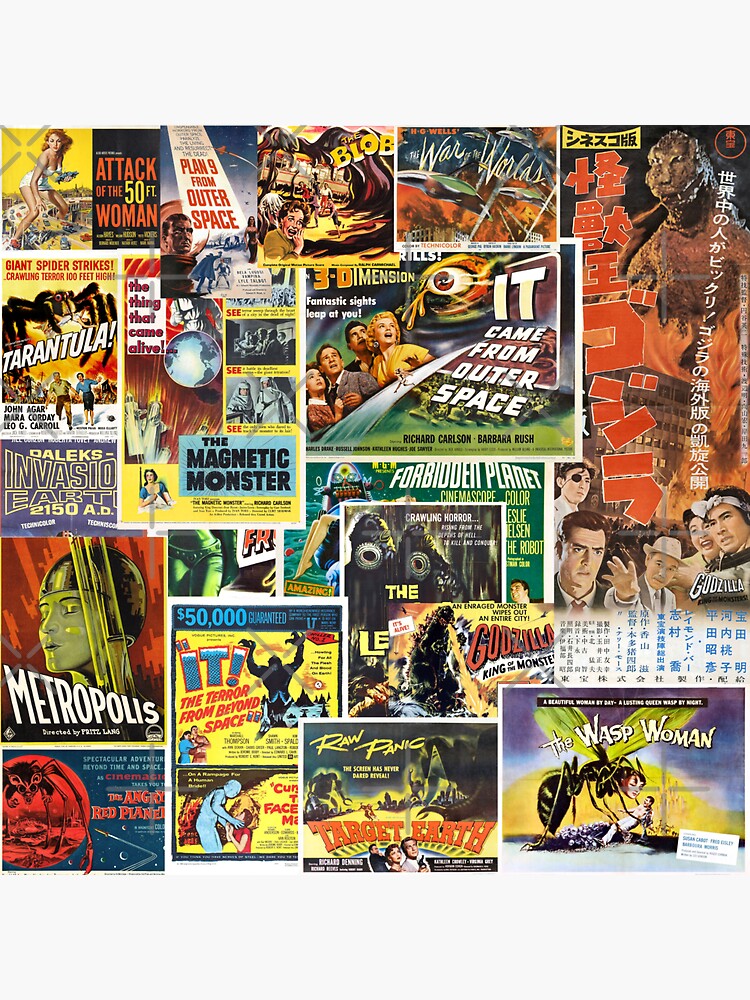The image is a detailed collage of vintage sci-fi and horror movie posters, predominantly from the 1950s. Arranged in a mosaic on a white background, the posters form a vibrant and nostalgic snapshot of mid-20th-century cinema. Dominating the top left corner is the iconic "Attack of the 50 Foot Woman," depicting a giant woman trampling over cars. From there, the collection cascades down to the bottom right, showcasing titles such as "It Came From Outer Space," with its eerie eye, and "The Wasp Woman," featuring a striking image of a woman transforming into a wasp-like creature. Among these, the original "Godzilla" poster is notable, complete with Japanese lettering, and "Forbidden Planet" commands attention at the center. The posters display a rich palette of colors, including reds, oranges, greens, yellows, and beiges, evoking a sense of their era's bold aesthetics. Each piece contributes to the overall theme of classic B-movie flair, punctuated by a shared style of dramatic illustrations and sensational titles.